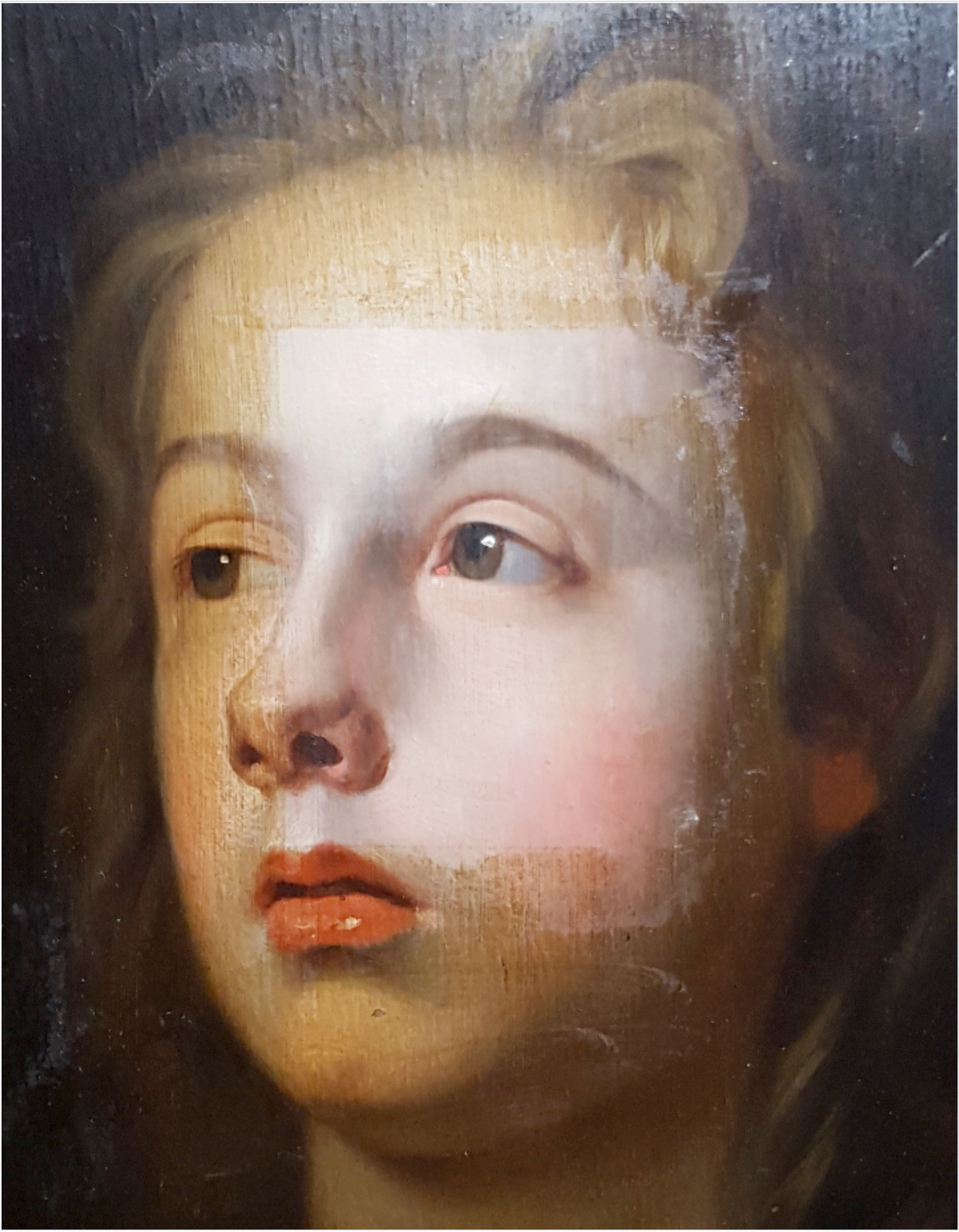The image is a close-up photograph of a worn and aged oil painting, depicting a young girl, possibly a teenager, gazing to the left. The painting appears to be in the process of restoration, evident from a clean, rectangular section near the top of her lip and forehead above her left eye. The girl's brown, messy hair frames a face marked by a pained, sad expression, and her red lips stand out against her otherwise yellowish skin tone, which appears more natural inside the restored square. The painting's surface reflects light powerfully, particularly at the top, revealing the texture of the actual canvas and the reflective nature of the oil medium. The subject, thought to be from the late 1800s, has white porcelain skin with slight scruff on the side, intensifying the timeworn feel of the artwork.